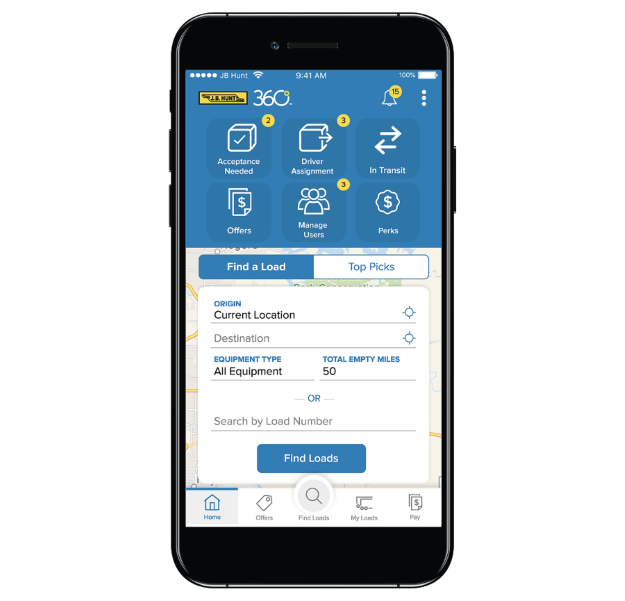A black smartphone is prominently displayed, with its screen showcasing a web application. The device features a front-facing camera, identifiable by the small circular cutout at the top. The screen is divided into distinct sections: the upper third adorned in a mid-tone blue, while the remaining two-thirds are predominantly white. In the background, there is a map, subtly visible.

The top section of the screen displays a heading labeled "360," accompanied by a notification bell icon on the right side, which has a yellow badge indicating 15 notifications. Directly below, four interactive boxes are presented, each with white text. They are labeled as follows: "Acceptance Needed," "Driver Assignment," "In Transit," and in a lower segment: "Offers," "Manage Users," and "Parks." 

Further down, options for finding loads are available, with prompts such as "Find a Load" or "Top Picks," allowing the user to enter various pieces of information. The "Find Loads" button stands out in blue with white text. At the bottom of the screen, navigational options are provided: "Home," "Offers," "Find a Load," "My Loads," and "Pay."